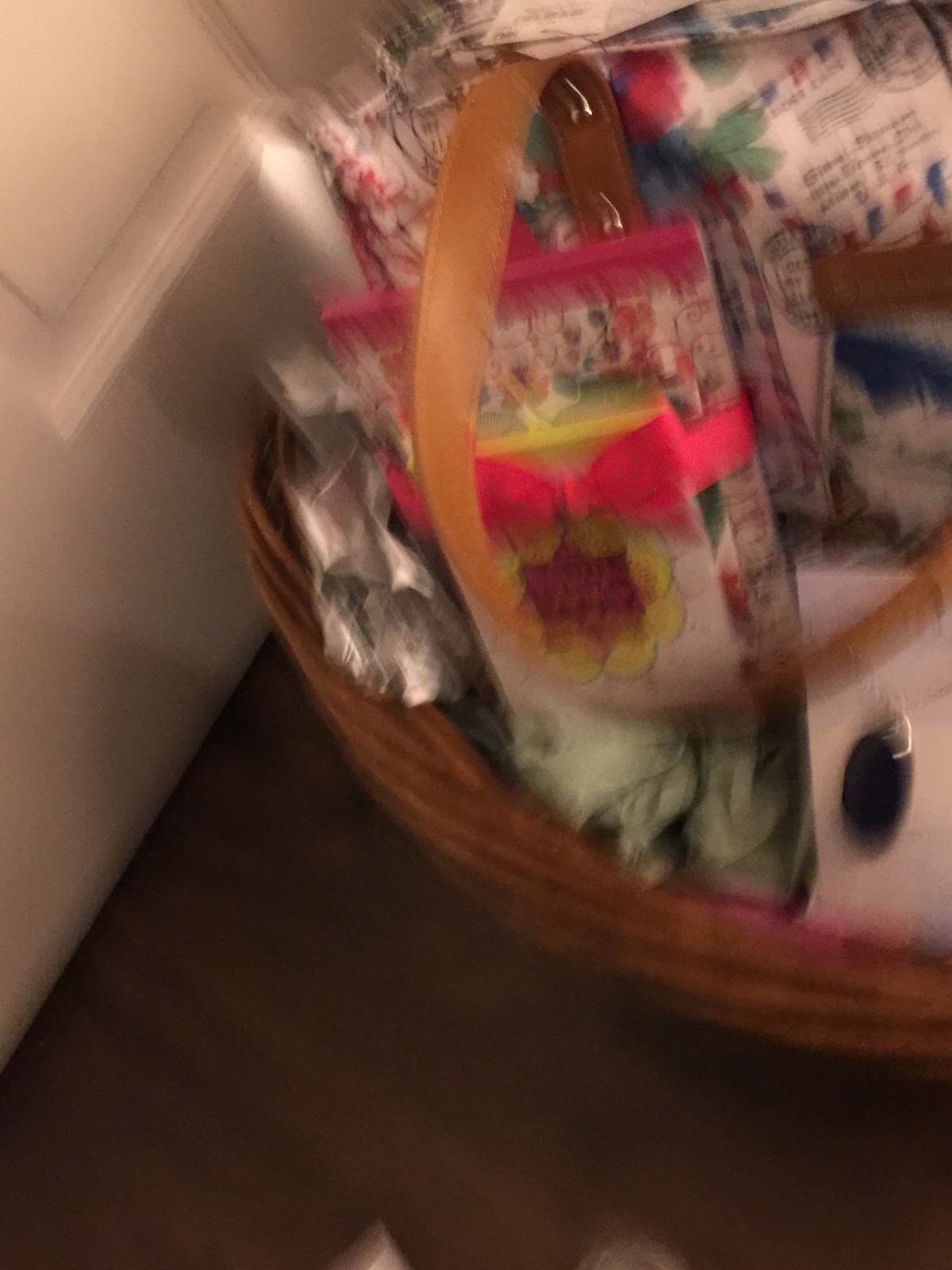This extremely blurry photograph depicts a scene from above, focusing on a woven wooden basket filled with various items. The basket is placed on a dark brown, wooden floor, near what appears to be a white door or wall, though the exact nature of this background feature is unclear due to the blurriness. Inside the basket, there are several indistinct objects, with some identifiable as a pad of stationery, a child-sized belt or possibly a dog leash, and a small square gift adorned with a red bow. Decorative crumpled paper in various colors, including a patterned paper with red, green, and black elements on a white background, surrounds the items in the basket. Despite the overall out-of-focus nature of the photograph, the wood grain of the floor and the weave of the basket are faintly discernible, along with a potential leather clasp hinting at the presence of a bag inside the basket.